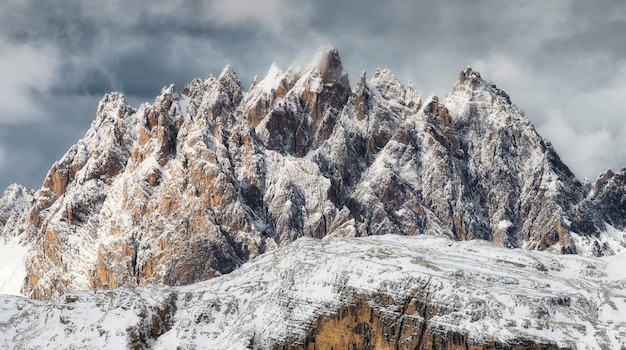The image depicts a barren, snow-covered mountain landscape with jagged, steep peaks that are a blend of gray and brown rock. The rocky surfaces, where not covered in snow, exhibit a rugged texture, and there is no visible vegetation. The snow appears thin and windswept, with its undisturbed, streaked patterns accentuating the cold and foreboding atmosphere. The sky above is overcast with thick, whitish clouds interspersed with darker gray ones, casting a bleak and inhospitable mood. The sharply pointed peaks resemble teeth or fangs, and the terrain ranges from potentially traversable lower cliffs to almost entirely intraversable high angles. The overall scene is stark and imposing, suggesting a remote and desolate wilderness.